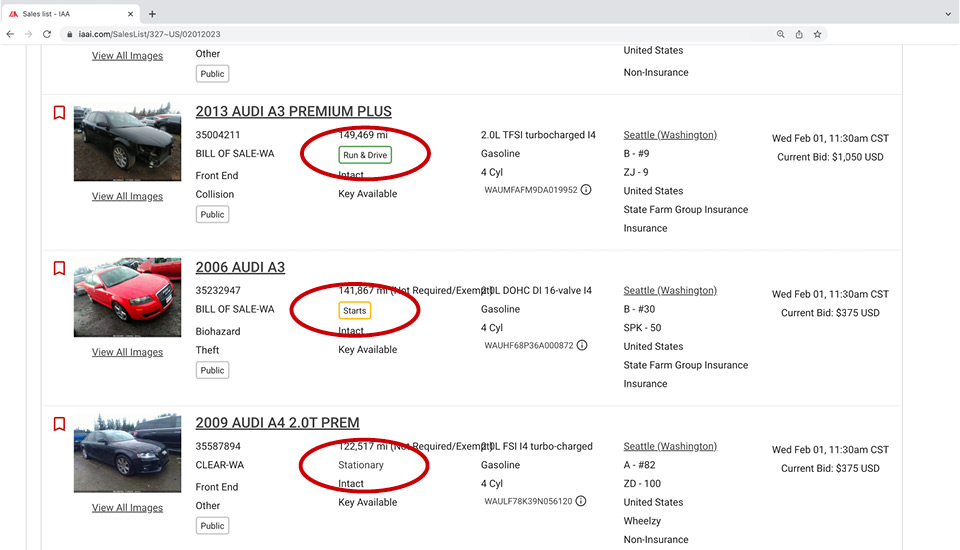This image is a screenshot of a company's sales list webpage. In the upper left corner, the website "Sales List IAA" is displayed, featuring a red logo to its left. Directly below, the search bar indicates the URL "IAAI.com/saleslist/327". The main section of the screenshot begins with options to view all images and filter by location, specifically "United States."

The list starts with a 2013 Audi A3 Premium Plus, along with an image of the vehicle to the left. The listing shows the car is being sold with a Bill of Sale from Washington and has a mileage of 149,469.

Below, a red 2006 Audi A3 is listed next with 141,867 miles on it and is also being sold with a Bill of Sale from Washington.

Finally, a black 2009 Audi A4 2.0T Premium is listed with 122,517 miles and the same Bill of Sale conditions from Washington.